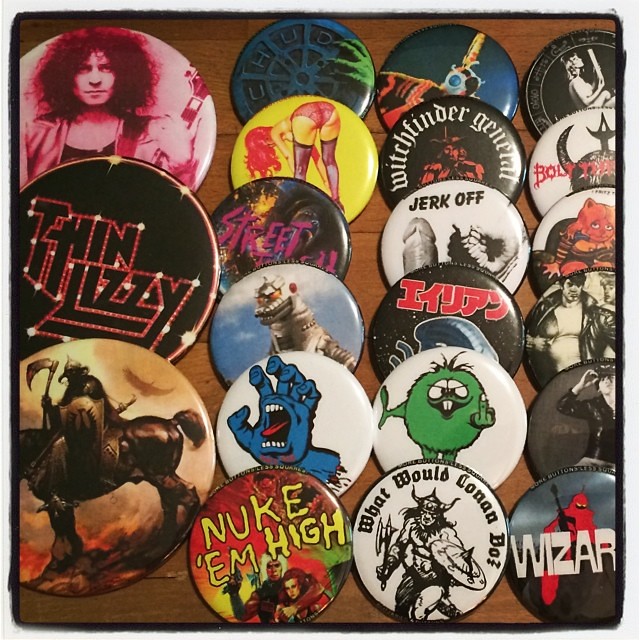The image depicts a collection of sarcastic and humorous pins laid out on a brown wooden table. The pins are mostly of the same size, though a few larger ones are arranged in a distinct column. The collection features an assortment of designs, including band references like "Thin Lizzy" and varied characters such as "Conan the Barbarian." One pin provocatively displays a green figure making a rude gesture, while another features an oddly intriguing image of a hand with an open mouth. The pins are vividly colored, showcasing shades of white, pink, red, yellow, green, blue, and more, adding to their eclectic and vibrant appearance. Despite the pins being spread out without a specific central alignment, the arrangement of six pins down and three across, with the bigger ones forming a separate column of three, is evident. The setting appears to be a casual indoor environment, possibly someone's personal collection displayed on a dresser.